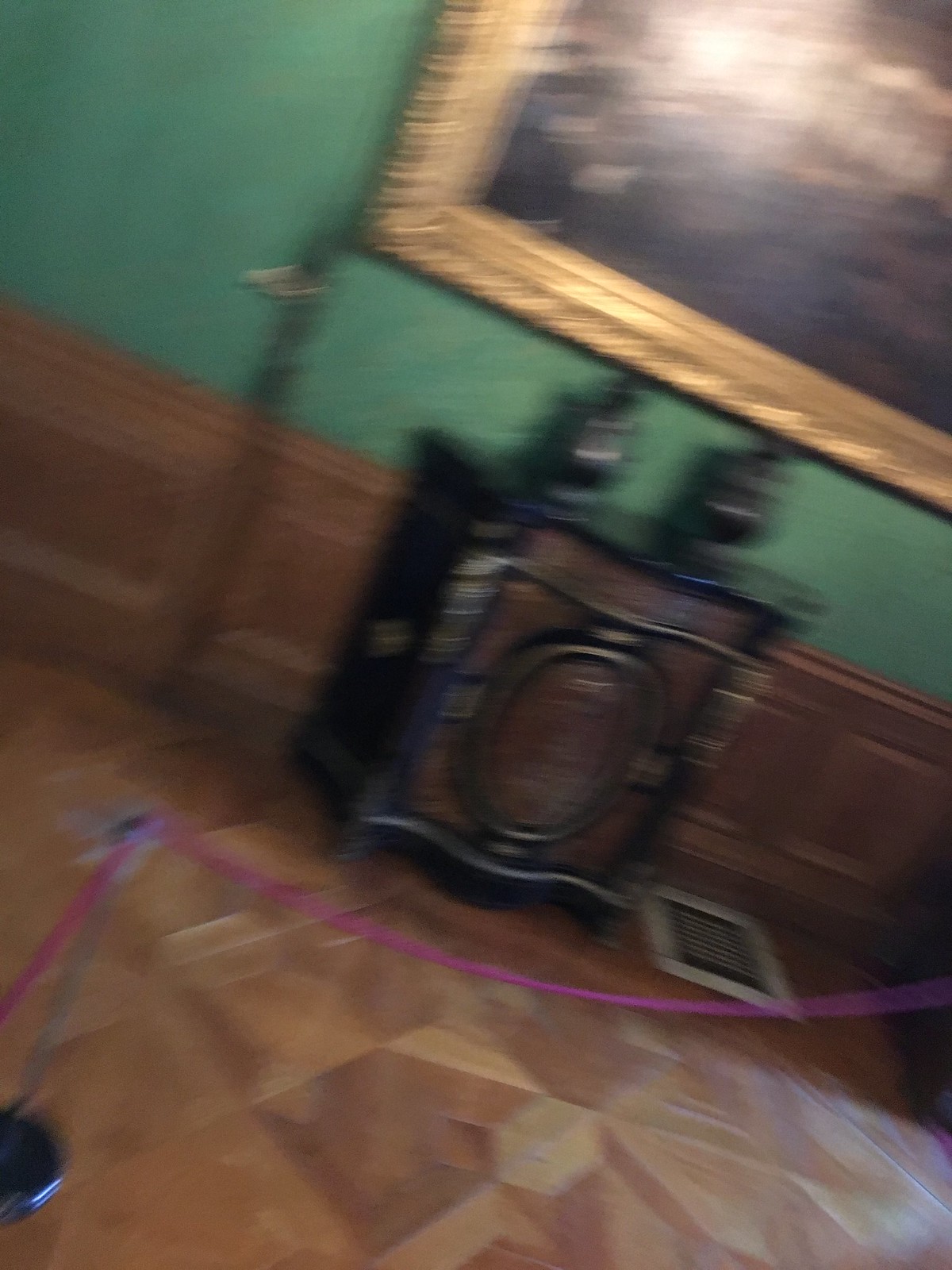This somewhat blurry photograph appears to have been taken inside a museum. In the foreground, there is a silver stanchion connected to a burgundy or magenta-colored rope that sections off a part of the exhibit area. The floor is crafted from mid-tone wood and features an intricate floral pattern etched into its surface. Part of a mid-tone brown wooden wall is visible, topped by a partially seen green upper wall. Against the lower wooden wall stands a piece of antique furniture, which is adorned in shades of black, gold, and brown. Two black objects are placed atop this furniture. Above these items, a large painting with a gold flake border hangs prominently. The painting itself is rendered in tones of gold, brown, and black.